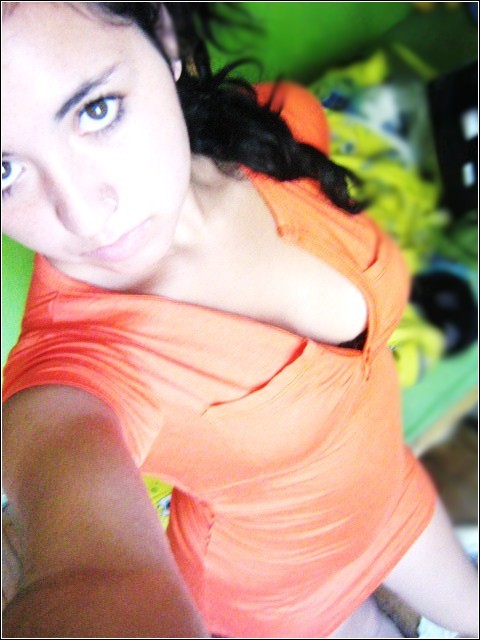The image is a selfie of a young Middle Eastern woman in her 20s with long black hair. She is wearing a short, vibrant orange dress that reveals her cleavage and a black bra underneath. Her hair cascades over her left shoulder as she looks directly into the camera, holding the phone with her right hand, visible in the lower left corner of the photo. The dress is quite short, exposing her legs in the lower right part of the image. The background appears chaotic with a green couch cluttered with various clothing items, although the details are blurry and indistinct. The woman's face is positioned near the top left corner of the frame, and the perspective of the shot looks down onto her torso, emphasizing her bright, colorful outfit against the messy backdrop.